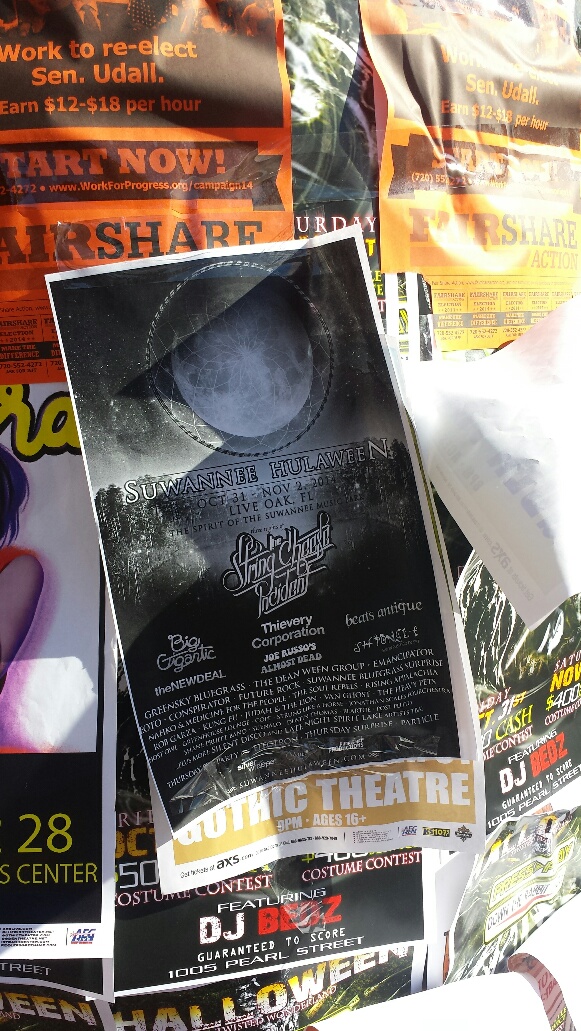This image captures a bulletin board plastered with an array of vibrant flyers promoting various events. Central to the display is a prominent black and gray flyer with a circular moon and star motif that announces "Suwannee Hulaween," a Halloween-themed music festival held in Live Oak, Florida, from October 31st to November 2nd, 2014. The festival features notable acts such as The String Cheese Incident, Big Gigantic, Thievery Corporation, Beats Antique, Joe Russo's Almost Dead, The New Deal, and Greensky Bluegrass, emphasizing a mix of bluegrass and jam band genres.

Surrounding the central flyer are additional posters, including one advertising a DJ event on Pearl Street, another promoting Airshare with a call to "Start Now," and a political flyer supporting Senator Udall's re-election campaign, offering wages between $12 to $18 per hour. The image, taken during the day, captures the intricate details of the flyers, with bright reflections and shadows highlighting their colorful designs against the backdrop.